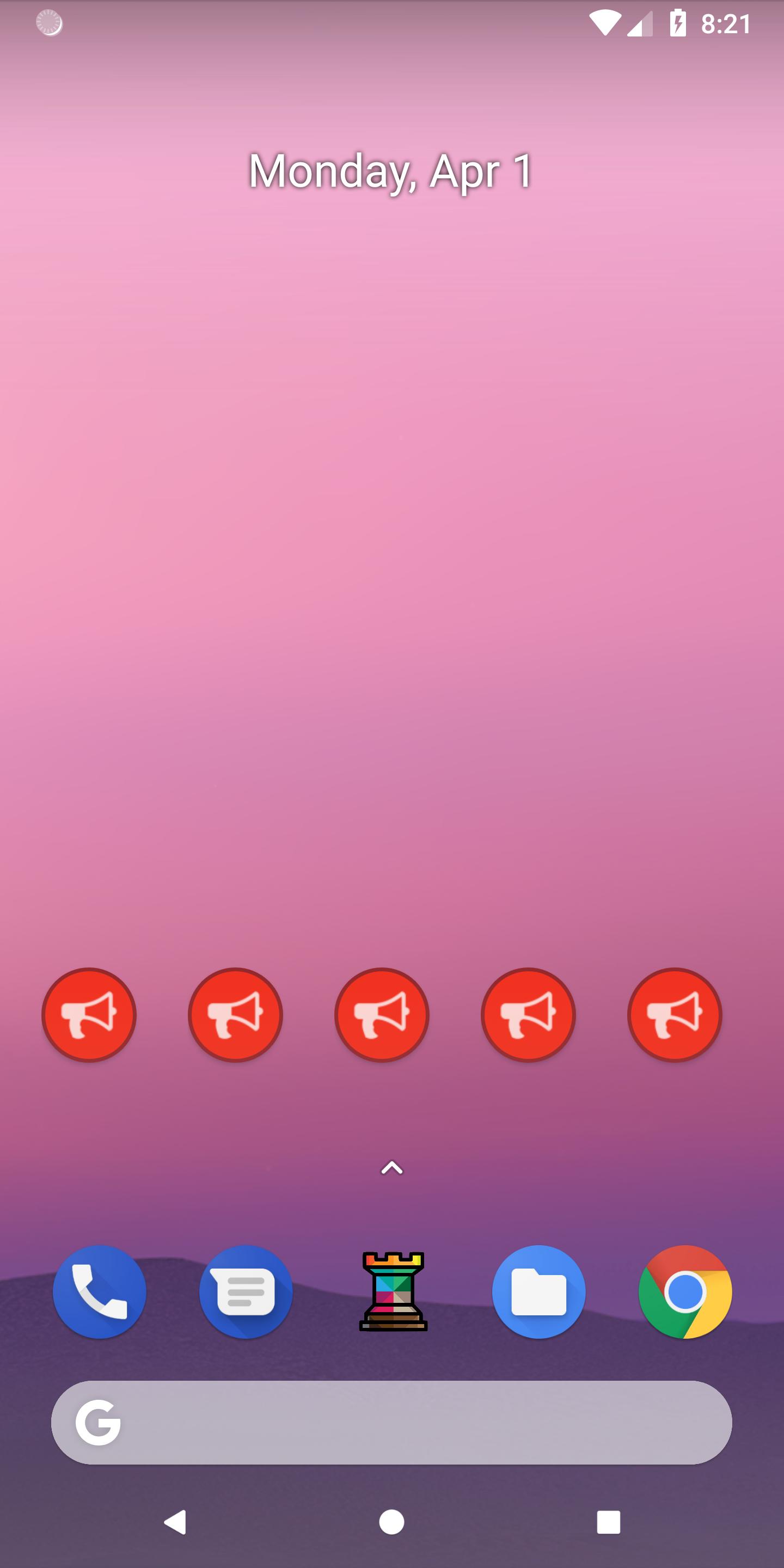This is a screenshot of a mobile phone's home screen. At the top of the image, a whitish-gray notification circle is visible, followed by a Wi-Fi signal icon, a battery icon without a percentage indicator, and a Wi-Fi strength symbol. The time displayed is 8:21 AM. Below this, the date "Monday, APR 1" is shown against a pink and purple wallpaper backdrop.

In the middle of the screen are five icons, each represented by a red circle with a white bullhorn symbol, followed by a white upward arrow underneath. Further below, there are several additional app icons:

1. A blue and white phone symbol inside a blue circle.
2. A blue and white text bubble icon inside a similar blue circle.
3. An icon resembling a chess pawn with a gold crown, colored in shades of teal, green, pink, tan, and brown.
4. A blue circle with a white manila folder icon.
5. The Google Chrome icon in red, gold, blue, and green.

At the bottom of the screen is a small Google search bar with a white "G" logo, accompanied by navigation icons: a white back triangle, a white circle (home button), and a white square (recent apps).

The image is of excellent quality, making each detail clearly discernible.